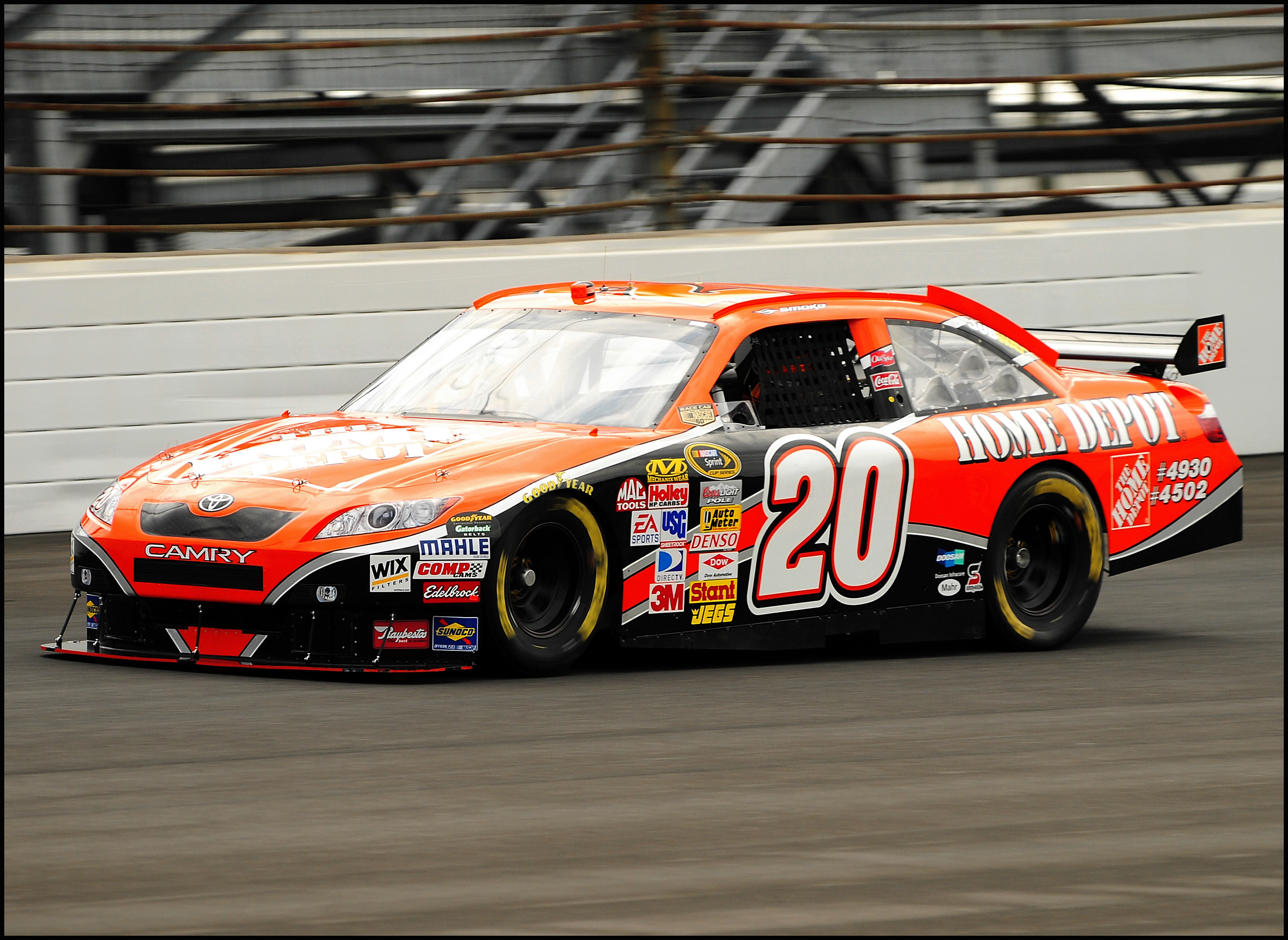The photograph captures a vibrant, professionally racing Toyota Camry on a gray asphalt track, seemingly in motion as indicated by the motion blur effect on its wheels. The car is predominantly orange, adorned with an array of sponsor logos and text, including prominent ones like "Home Depot," "Camry," "Wix," "Comp," "Denso," and "3M". The number "20" is prominently displayed in white on the left driver-side door, accented with black and orange outlines. The front of the car showcases the "Toyota Camry" logo, while the "Home Depot" branding is prominently placed on both the hood and the rear side. The lower sections of the car feature dark bands with white borders, adding to its dynamic aesthetic. The backdrop features a white-painted brick fence and no visible people, highlighting the car as the central focus of this action-packed shot.